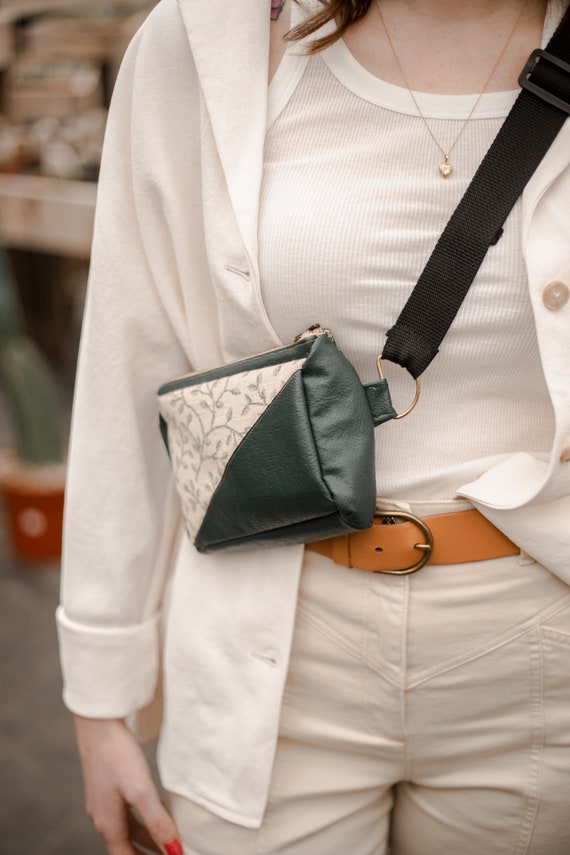The photograph features a woman, though her face is not visible, as the image captures her from the neck down. She has fair skin, possibly indicating she is Asian or Caucasian. Her outfit is predominantly off-white, consisting of an off-white tank top, pants, and a matching off-white jacket with sleeves rolled up to her wrists. The jacket is slightly asymmetrical, with the right side partially tucked in and the left side untucked and unbuttoned. She accessorizes with an orange belt and a delicate gold necklace with a heart or penny pendant.

She is also carrying a sizable pocketbook with a combination of white and green, featuring a floral pattern and a distinctive white triangle design with leaves and smaller twigs embroidered into it. The bag is equipped with black straps slung over her shoulder. Noteworthy details include her red fingernails, which add a pop of color to her monochromatic ensemble. The background suggests she is in a public space, possibly a market, due to the blurred objects and shapes visible. She is facing the camera, but neither her head nor her feet are shown in the image.